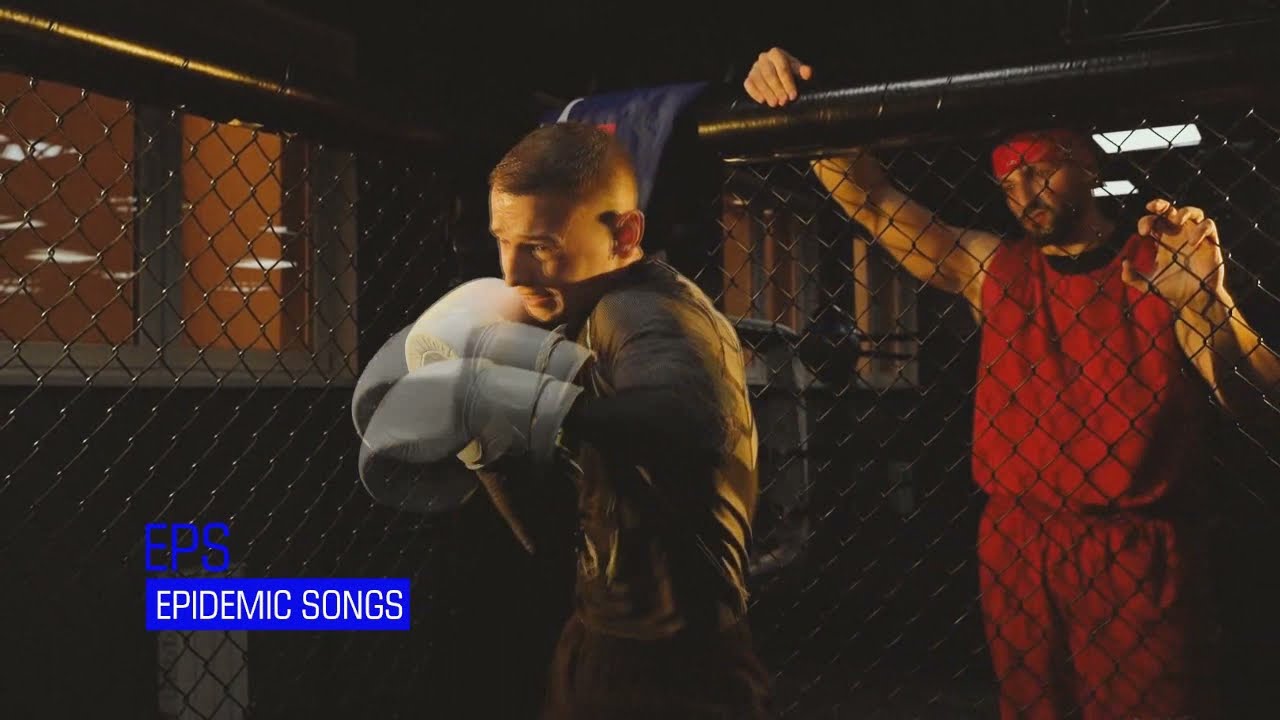The image appears to be a stylized, colorful scene, possibly from a video game or music video. In the bottom left-hand corner, “EPS” is displayed in bold blue text above a blue box with the words "epidemic songs" written in white. The central focus of the image is a man inside a black chain-link fence, who appears to be a fighter. He is wearing a black outfit consisting of a long-sleeve shirt and pants, with white boxing gloves raised above his head, ready to strike. His hair is short, and he has a light skin complexion. Behind the fence, towards the right, another man, similarly light-skinned, stands with his right hand on top of the fence and his left hand grasping the chain link. This individual is dressed entirely in red, including a sleeveless red shirt, red pants, and a red bandana on his head. He is looking intently at the fighter inside the cage. The background features a row of windows and some white lights in the upper right-hand corner.